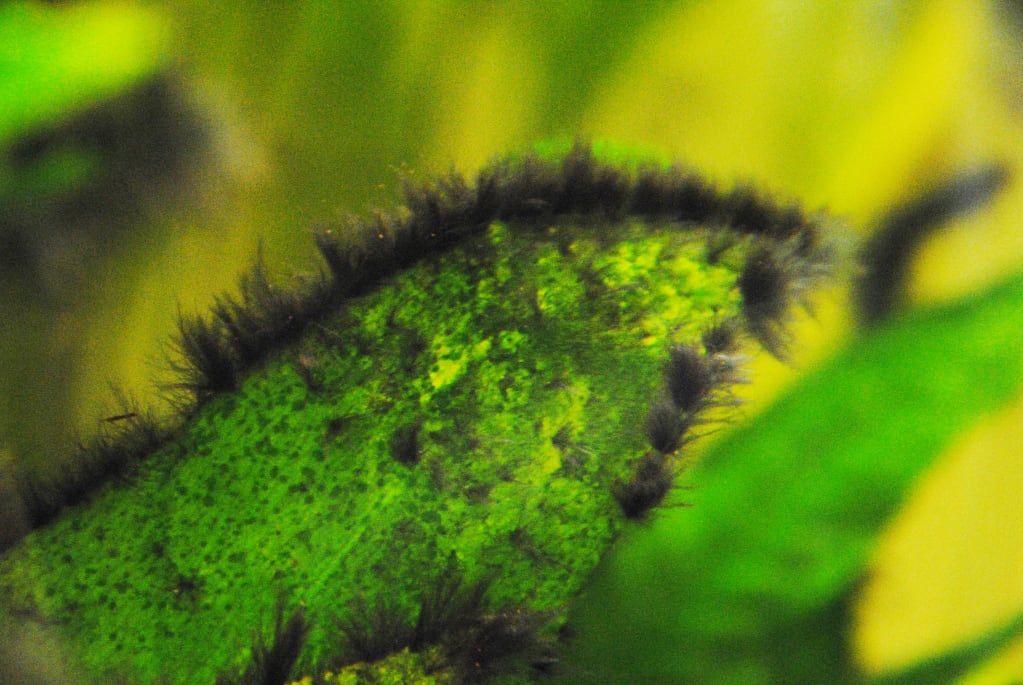The image showcases a close-up of a green, triangular, and pointed leaf that is notably fuzzy and covered in short, black hair-like structures, which may be natural or indicative of some type of fungus or infestation. The leaf extends from the bottom left towards the center of the image and is partially out of the frame, suggesting a zoomed-in perspective. The background is blurred, featuring yellowish-green hues and indistinct plant material, providing a contrasting backdrop to the sharply focused, peculiar texture of the leaf. The black hairs are distributed along the edges and scattered across the leaf's surface, giving it a distinctive, almost fur-like appearance that raises questions about its condition or species.